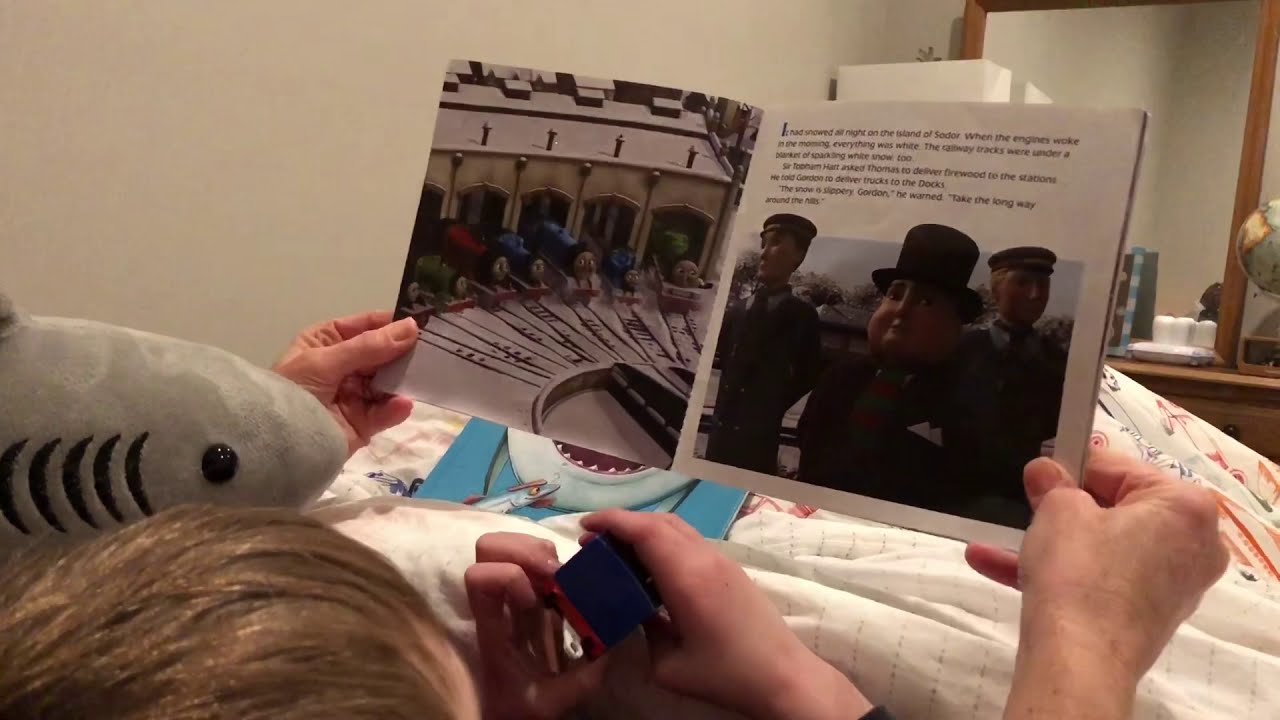In the image, a warm indoor setting unfolds depicting a moment of storytime shared between an adult and a child. Centered slightly off to the right, an open book bathed in blues, reds, and greens hints at colorful illustrations, despite its text being too small to read. Below it, part of a blue-covered, closed book peeks into view. To the bottom left, the top of a child's brown-haired head is visible, with tiny hands suggesting engagement in the narrative. Above the child, a gray plush shark with black gills and a steely eye hovers, adding a playful touch. The adult’s hands, likely part of an unseen parent's arms, hold the book mid-story. In the background, a globe adorned in yellow and blue tones sits below a mirror framed in light brown wood, both in the top right corner. The varied colors of white, gray, black, brown, red, blue, and silver, along with the intimate arrangement, evoke a cozy evening or nighttime reading ritual, capturing the serene essence of bedtime storytelling.